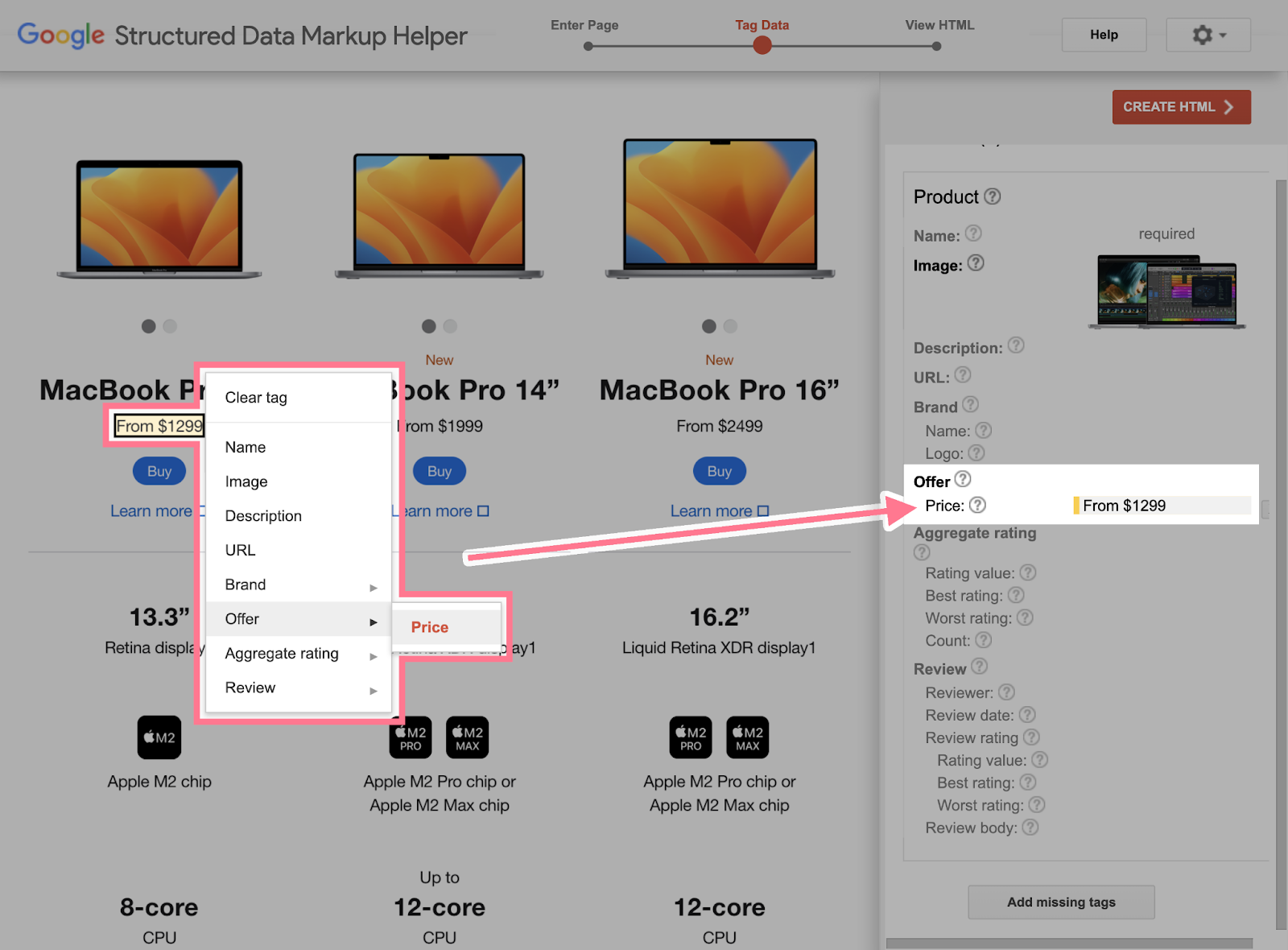The image depicts a Google landing page specifically designed for the Structured Data Markup Helper tool. The interface is slightly obscured by a darker overlay due to an open pop-up window in the top left-hand corner. 

At the top of the page, the Google Structured Data Markup Helper title is prominently displayed. "Google" is presented in the company's iconic multi-colored logo, while "Structured Data Markup Helper" is in black text. To the right of the title, there is a slider bar. The left side of the slider reads "Enter Page," and the right side reads "View HTML," with a red circle at approximately the midpoint, indicating the current selection. Above this bar, the label "Tag Data" is visible.

Further right, there is a white box with a gray border around it, containing the word "Help" in black text. Adjacent to this box is a settings icon accompanied by a dropdown arrow, also encased in a similar white box with a light gray border.

The main section of the screen features a white background showcasing three options for MacBook purchases. Each entry is illustrated with an identical image of a laptop, which increases in size correlating with larger screen sizes. Below each laptop image, there are detailed descriptions including pricing information. Each option also has a small blue button labeled "Buy" in white text. Toward the right side of the screen, a price of $1,299 has been selected by the user.